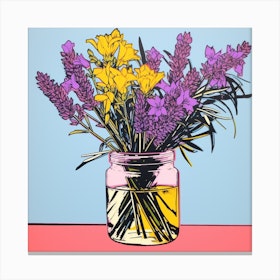The image is a tightly cropped, roughly square cartoon graphic art style depiction of a bouquet of purple and yellow flowers in a clear, wide-mouthed mason jar. The jar, filled with water up to about three-quarters of its height, shows dark yellow on one side and lighter yellow on the other. The stems within the jar are mostly black, with some appearing greenish-black. The mason jar’s top portion is subtly tinted pink. The flowers include long purple blooms interspersed with clusters of yellow flowers, and some larger singular purple flowers. Green foliage complements the bouquet. The background transitions from a pale baby blue at the top to a thin strip of pink at the bottom, giving the impression of the jar sitting on a salmon-colored surface. The image contains no text or artist’s signature.